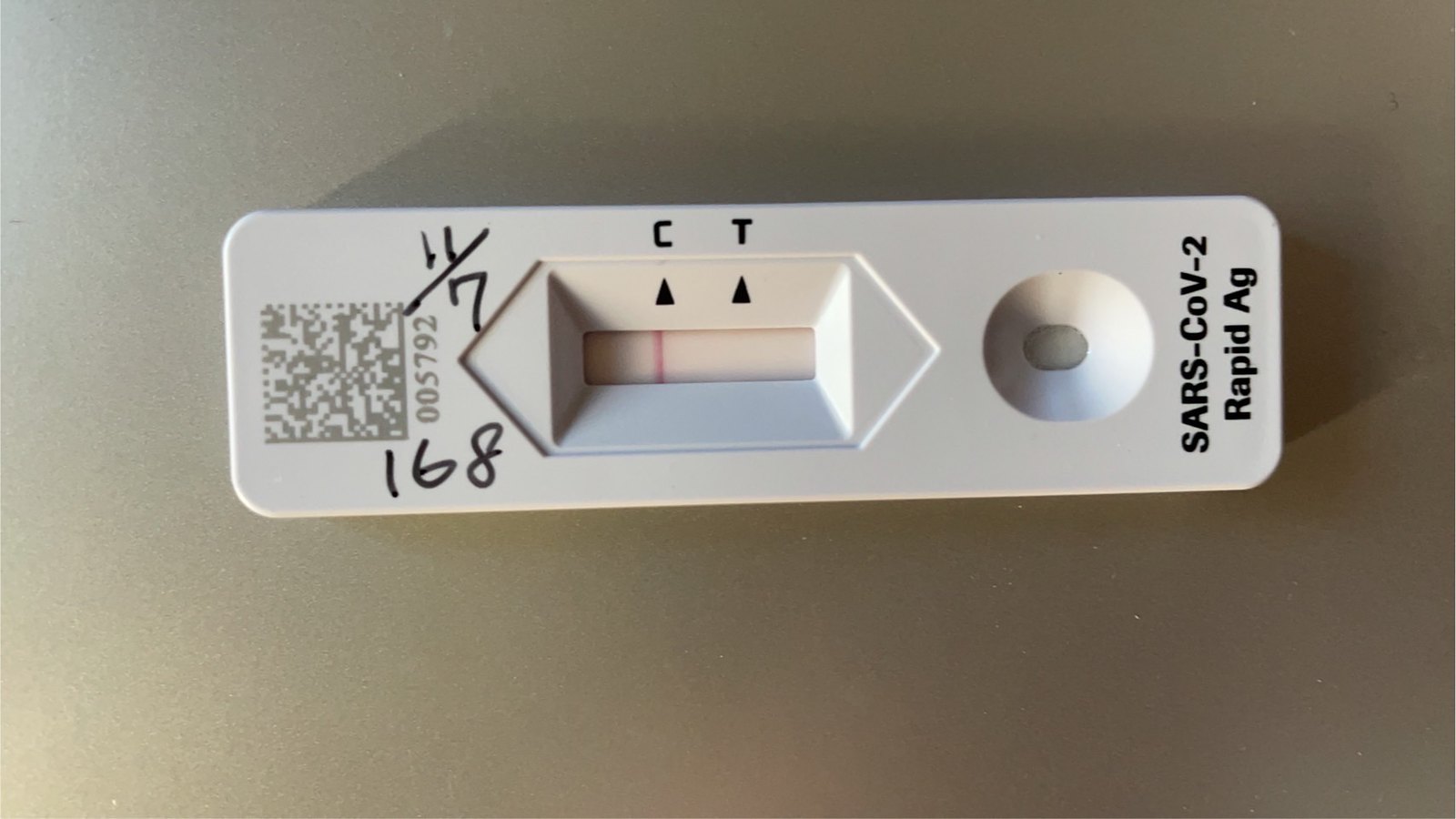This image showcases a SARS-CoV-2 Rapid Antigen (AG) test kit, lying horizontally on a brown background. The test kit features a clear rectangular window with a pink line visible in the "C" section, indicating a test result. The window is flanked by small arrows and labeled with "C" and "T" markers on either side. The kit includes a circular area, likely containing the test pad, positioned near the bottom. Below the test kit, the text "SARS-CoV-2 Rapid AG" is printed. Additionally, there is a QR code marked with the number "005792" underneath, and handwritten annotations including "11/7" and "168" in permanent marker. The image lacks any key or chart to interpret the test results as positive or negative.